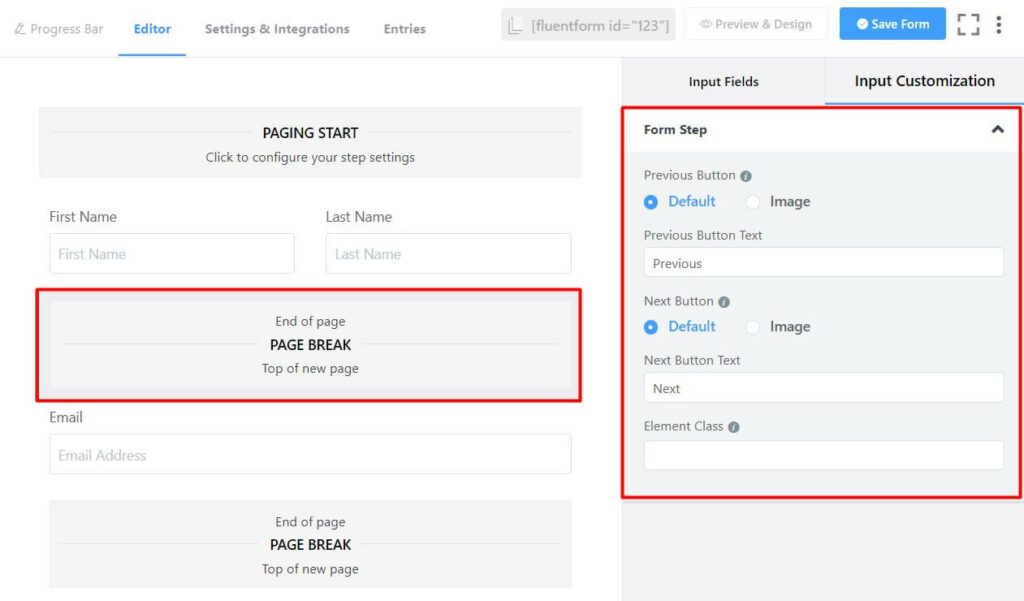This image captures a detailed screenshot of a technical customization page designed for configuring a step-by-step form setup. At the top of the screenshot, there is a progress bar, along with icons for editor settings and integrations, next to entries for the Fluent Form ID (123) and a "Save Form" option. The page features a variety of input fields, including text boxes for entering first and last names, and an email address, all of which are currently blank. There are multiple buttons for form navigation and setup, along with labeled sections for "page break," "top of new page," and "end of page." On the right side, inside a red square, there are default settings and images, as well as a "Next" button and configuration options for the next element class. This screenshot appears to be a specialized interface for web developers or webpage designers, providing a complex but well-labeled environment for entering and organizing data necessary for form creation or other technical setups.